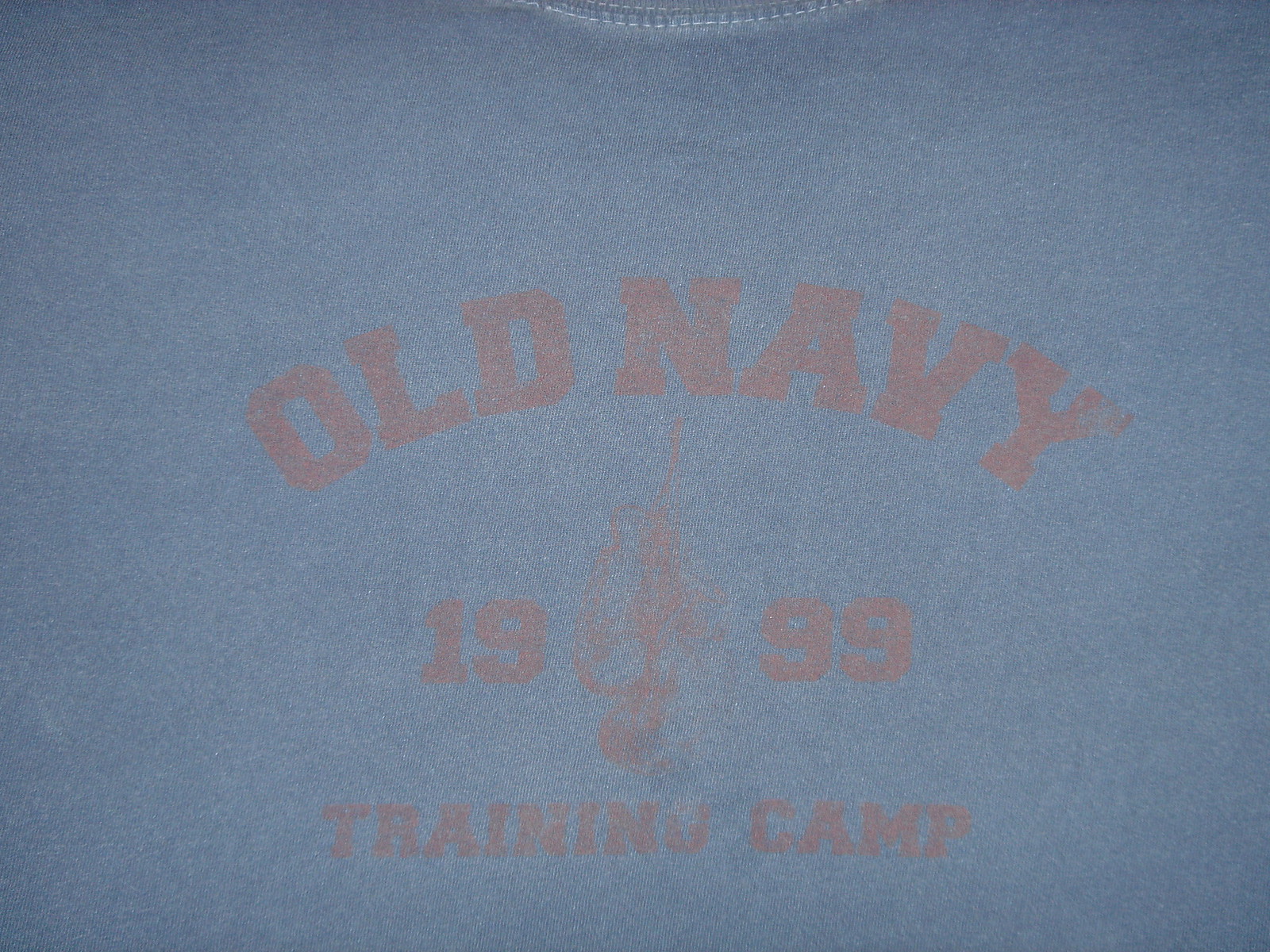This image features a close-up of a light-medium blue t-shirt, primarily showing the chest area. The shirt is adorned with white stitching around the collar, which is partly visible in the picture. A screen-printed logo sits in the center, characterized by a slight arch formation where the text curves upwards in the middle and slopes down towards the edges. The logo is in a faded orange color and reads "Old Navy" in capital letters. Below this, there are the numbers "19" and "99" separated by a heavily faded image that appears vaguely like a cat. Underneath these elements, the smaller, also faded text reads "training camp." The overall condition of the prints suggests significant wear, adding to the nostalgic appeal of the t-shirt.